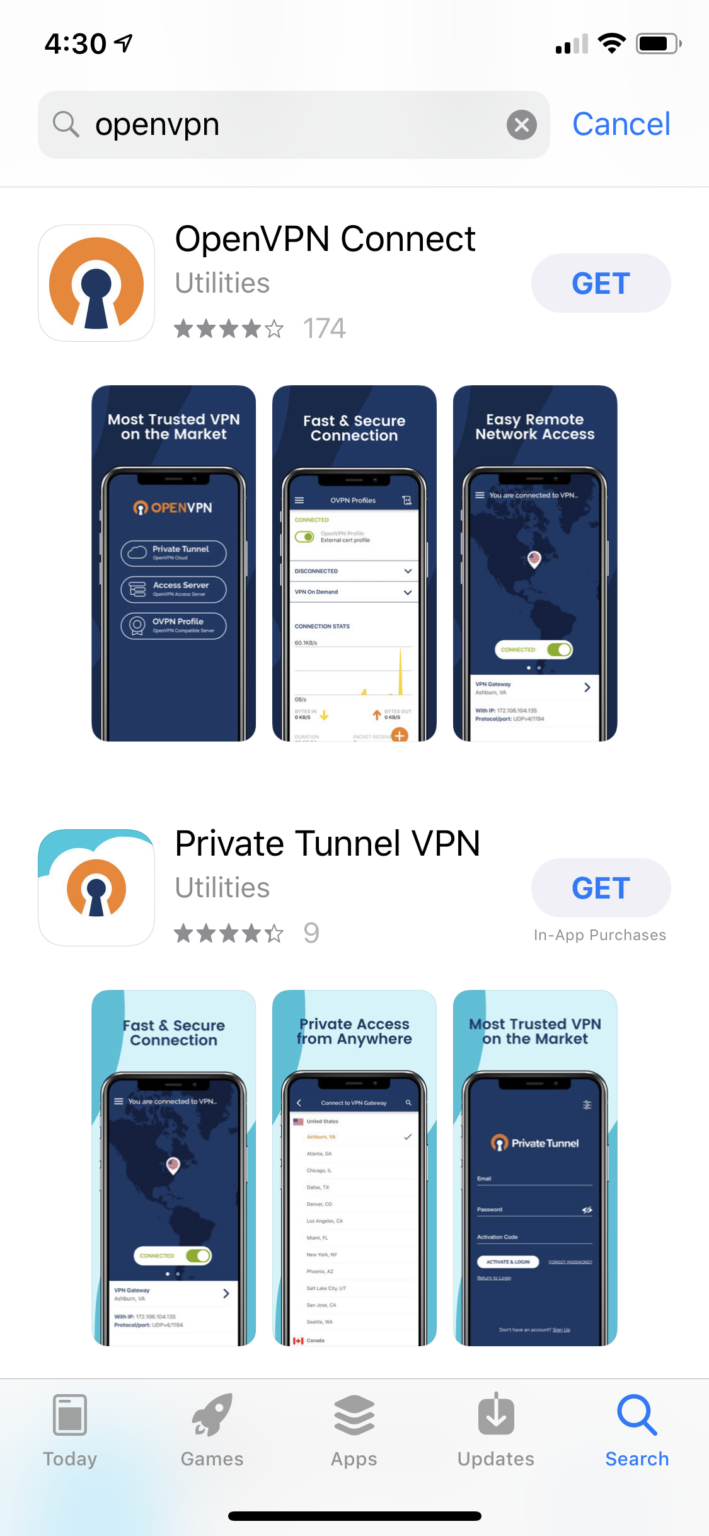The screenshot shows a smartphone screen with the current time displayed as 4:30. The device has 2 out of 4 bars for cellular signal, a full Wi-Fi signal, and approximately 80% battery life. At the top is a search bar with text that reads "OpenVPN" alongside a magnifying glass icon. An 'X' icon and a 'Cancel' hyperlink are positioned to the right of the search bar, with a light gray line below them.

Below the search bar, a square logo features a partial orange circle with a keyhole at its bottom. The text "OpenVPN Connect Utilities" is displayed beside the logo. A gray button labeled "Get" is visible in blue text in the middle. This app listing has a rating of 4 stars based on 174 reviews. Three smartphone screenshots, too small to be clearly read, are shown beneath this information.

Further down, another icon appears, resembling the aforementioned logo but set against a blue sky with clouds. This icon is for "Private Tunnel VPN Utilities," which also has a 4-star rating but with just 9 reviews. Similarly, three small screenshots are displayed below this app description.